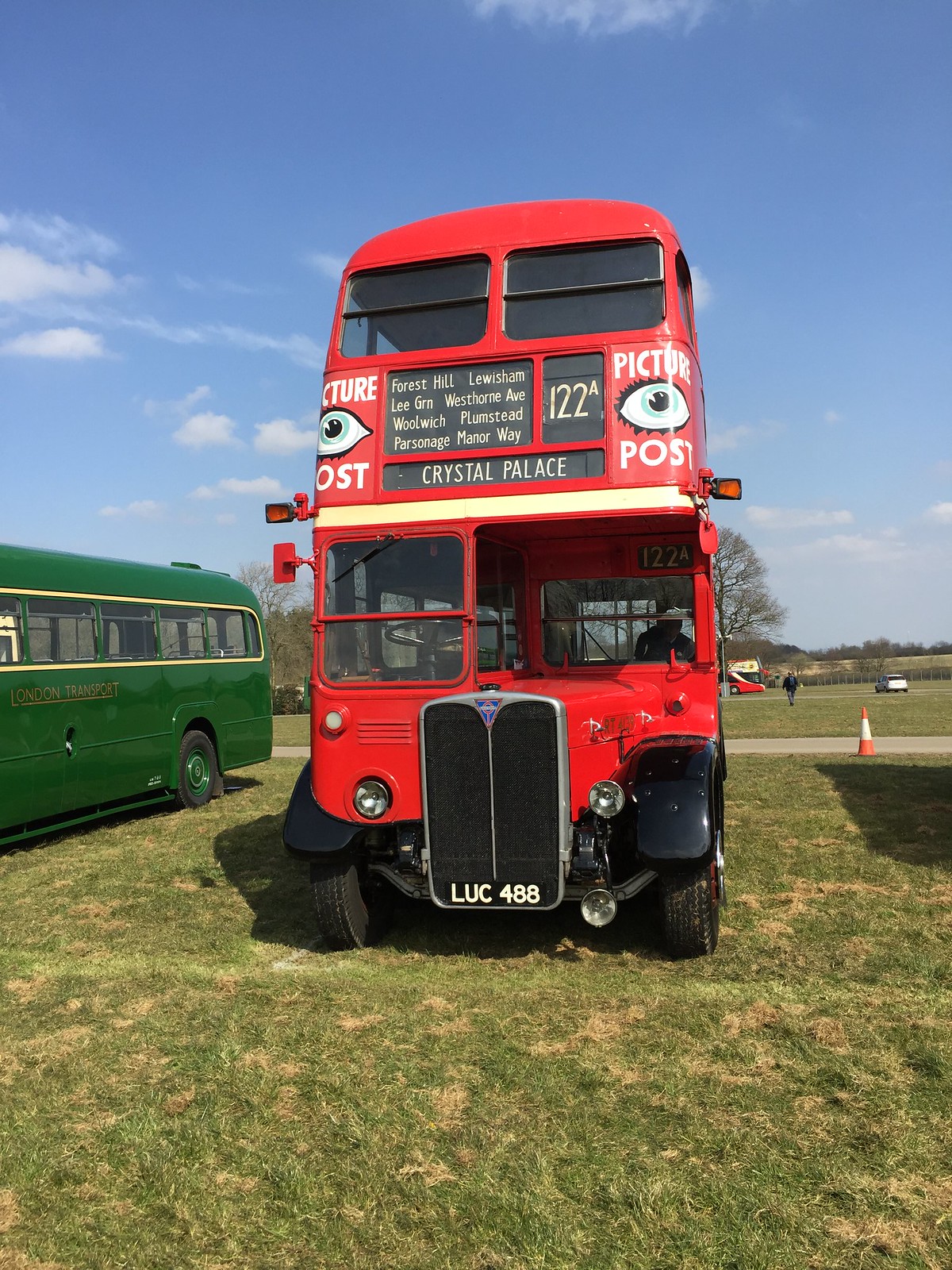The photograph captures a vibrant scene on a crisp, clear day with a predominantly blue sky and a few wisps of clouds. It showcases an old, red double-decker bus standing in a grassy field, possibly at a vintage bus meetup. The bus, designated as route 122A to Crystal Palace, has a distinctive, nostalgic charm with its very old-style front radiator adorned with a plate reading LUC488, and playful painted eyeballs above the driver’s alcove with a “Picture Post” sign in between. The driver’s area is recessed, creating a cozy nook at the front of the bus. To the left, a deep green single-story bus with green wheel rims and beige window trim stands in contrast. The background features more buses, including a distant red and white one, as well as a blacktop road and parked cars, suggesting a broader gathering. A person is seen walking towards the camera near a yellow traffic cone, adding life to the tranquil, yet visually rich outdoor setting.